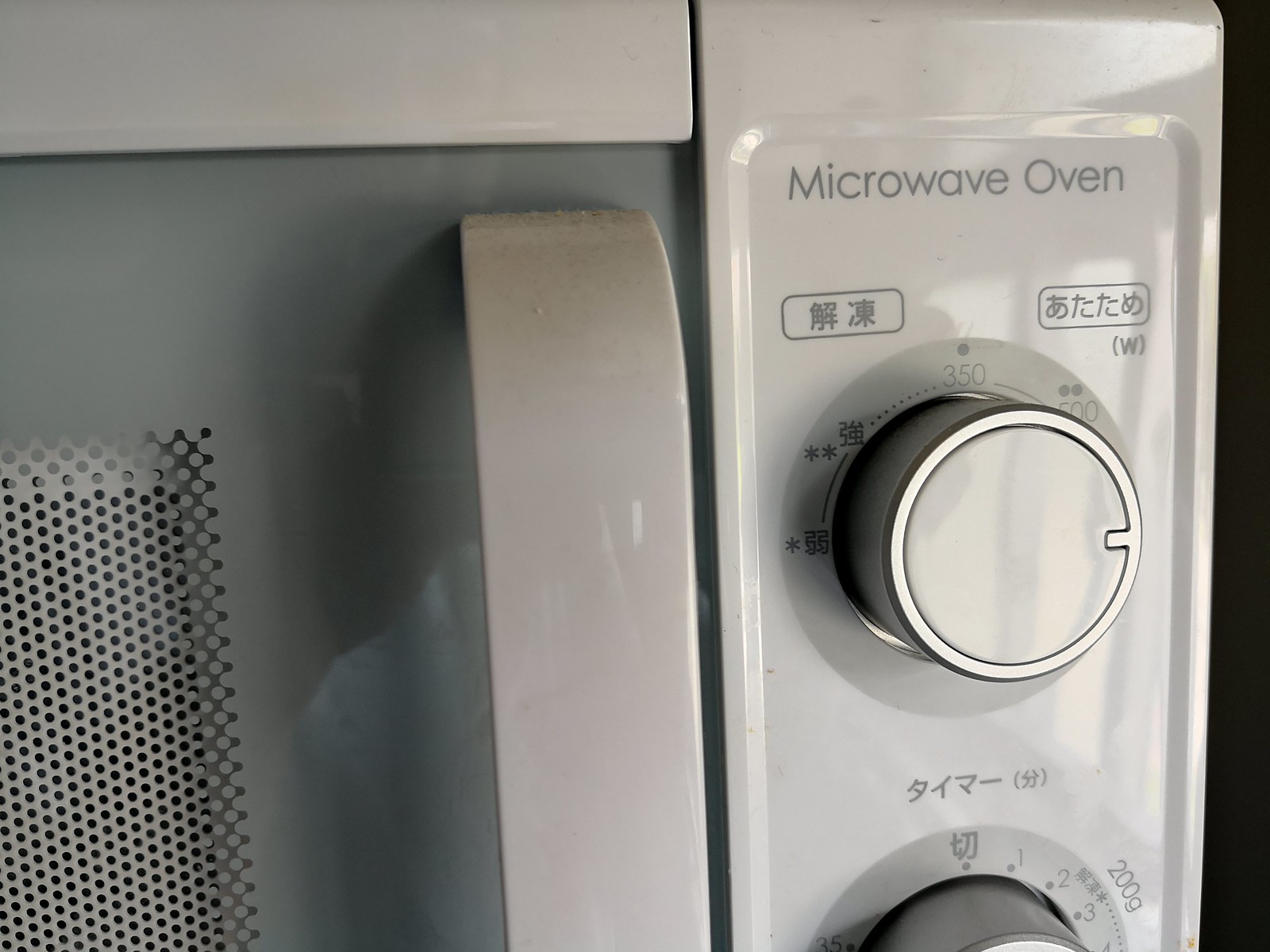This is a close-up color photograph of the upper right-hand corner of a microwave oven. The microwave features a white vertical handle centered in the middle of the image, reflecting light and partially showing the surrounding environment. The door of the microwave is gray with a perforated grid pattern allowing a view into the cooking chamber. The right side of the image showcases the control panel, which is predominantly white. At the top of the panel, in gray text, it reads "microwave oven." Beneath this text, there are two rectangular sections of Chinese or Japanese writing. Following that, there is a prominent silver knob with markings indicating the numbers 350 and 500, along with dots and lines guiding these settings. The bottom of the image reveals the upper portion of a secondary knob, also accompanied by Asian characters and numbers like 1, 2, 3, and 200G around its circumference. The entire microwave, with its reflecting handle and sunlit panel, exhibits a clean and functional design indicative of standard microwave ovens.